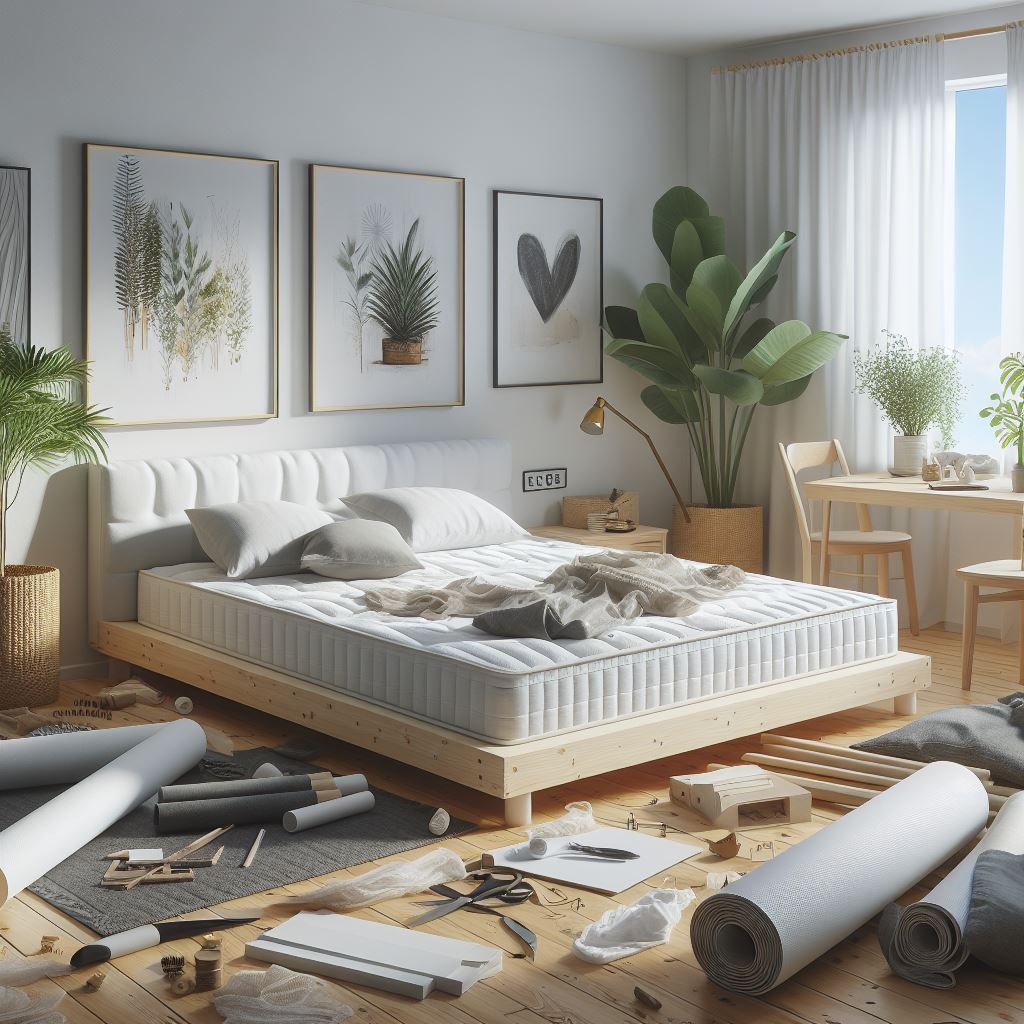This is an image of a bedroom in the midst of being assembled or renovated, displaying a blend of earthy tones and slight disarray. In the center of the room sits a king or queen-sized bed on a wooden frame with a headboard, topped only with a mattress. The bed is unmade, featuring two white pillows, a smaller gray pillow, and crumpled sheets towards the bottom. The wooden floor is scattered with various items, including cylindrical rolls and scraps, suggesting ongoing work or decoration. 

Adorning the back wall above the bed are three picture frames—two featuring plant illustrations and one with a black heart. To the right of the bed is a light-colored wooden table flanked by two wooden chairs, both bearing green plants on top. The room also houses a big green plant to the left of the bed, accompanied by a smaller plant near the corner. A dark gray rug lies to the left of the bed, adding contrast to the wooden floor.

Natural light filters through a window with partially open white drapes, enhancing the room's airy, natural ambiance. An earthy, minimalistic aesthetic is completed by the presence of a lamp and a clock on the wall, contributing to the overall sense of an inviting yet unfinished living space.